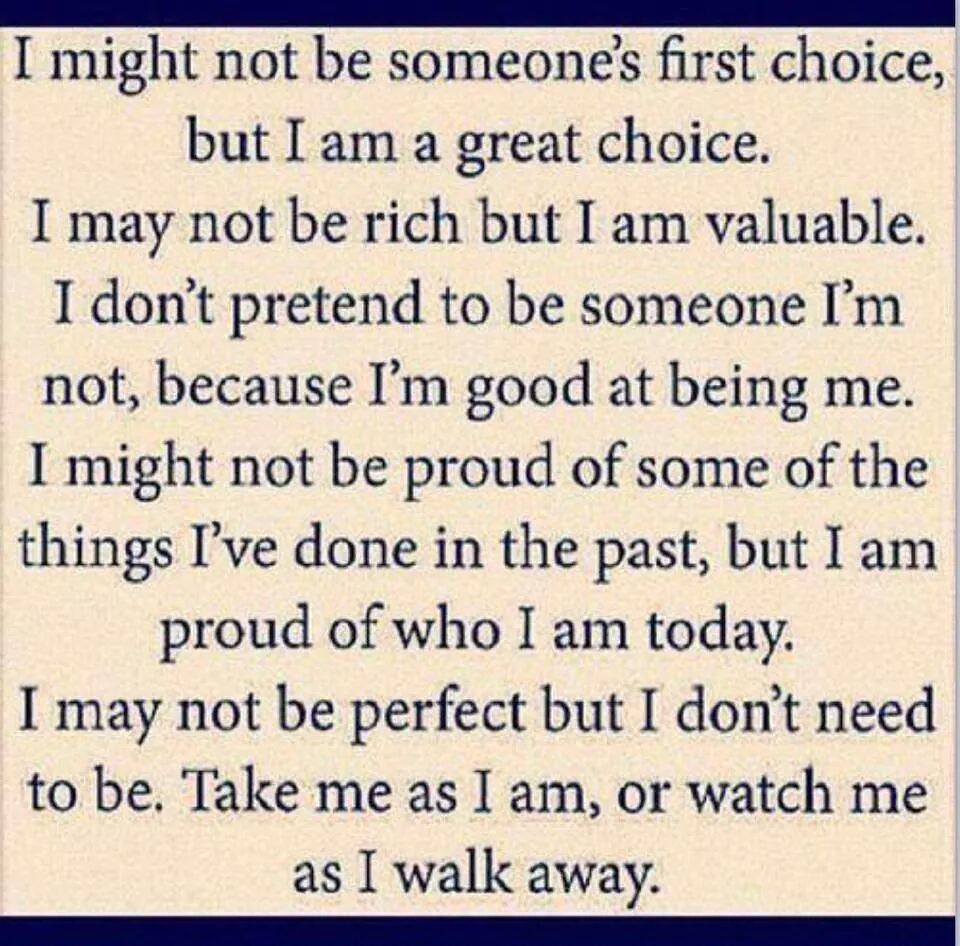This is an old, likely digital, image featuring an inspirational quote rendered in blue text against a yellowish-white, off-white background. The rectangular image has a distinctive blue border at both the top and bottom edges, with no borders on the left and right sides. The quote reads: "I might not be someone's first choice, but I am a great choice. I may not be rich, but I am valuable. I don't pretend to be someone I'm not because I'm good at being me. I might not be proud of some of the things I've done in the past, but I am proud of who I am today. I may not be perfect, but I don't need to be. Take me as I am or watch me as I walk away." The text is affected by noticeable JPEG artifacting, indicating that it is a low-resolution, highly compressed image. This could either be due to the image being from an older digital era or because it has been repeatedly saved and shared over time. Although the image appears low-res, it carries a strong message, making it ideal as a social media post, profile picture, or phone/computer screen background, but not something likely to be framed and hung on a wall.